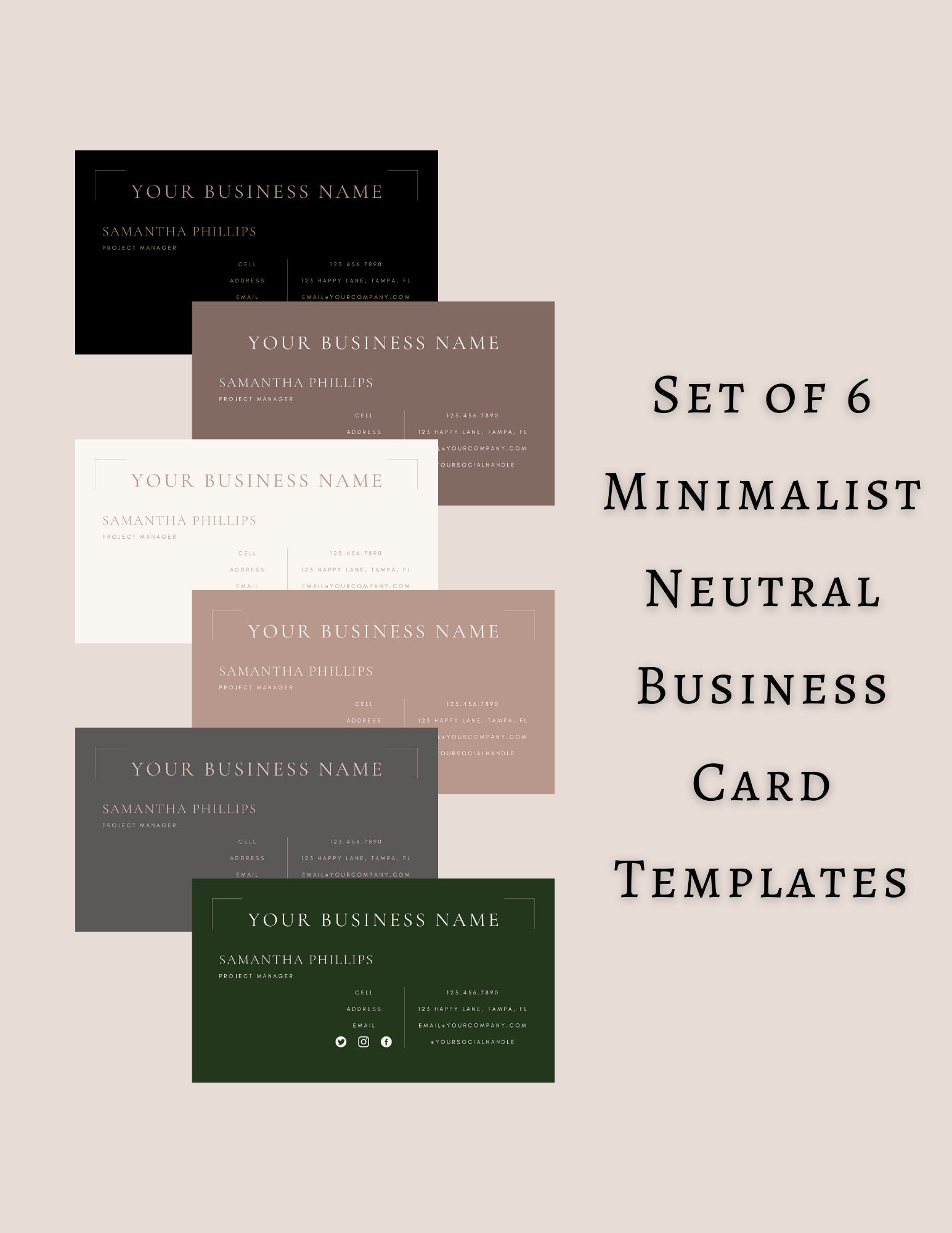The image is a promotional graphic for a set of six minimalist, neutral business card templates showcased on a very light pinkish gray background. The image mimics a website screenshot where users can customize business cards. On the right-hand side, in bold black text, it reads "Set of Six Minimalist Neutral Business Card Templates." The core design features six business card variants arranged in a staggered pattern from top to bottom, each displaying the heading "Your Business Name" with generic contact details. The background colors of the cards are distinctly different, proceeding in order from black, brownish-beige purple, white, dusty rose pink, gray, to a deeper evergreen. These cards exemplify various layout options for a business named "Your Business Name."